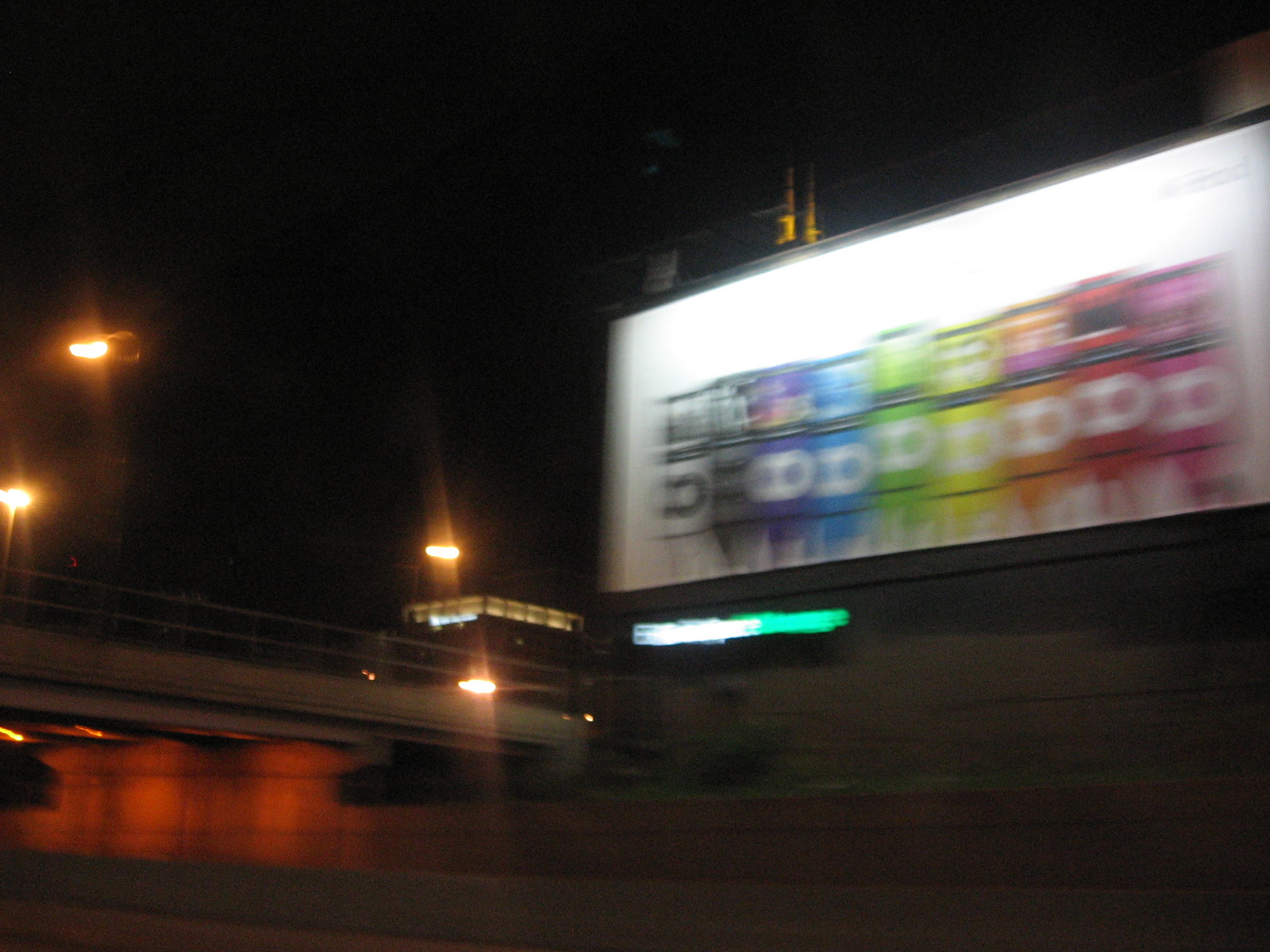This nighttime photograph showcases a billboard in an urban landscape. The image has a slight motion blur and is somewhat out of focus, rendering some details hazy. The scene features a central gray-colored wall with a hint of brown tones, serving as a textured road divider. A bridge with a matching gray hue crosses over this divider. Below the bridge, the wall glows warmly with an orange tint, illuminated by street lights. In the distance, yellow street lights add to the urban ambiance. Positioned in the upper right-hand corner, the billboard stands out with a stark white background adorned with a vibrant, rainbow-colored pattern. The colors transition sequentially through white, black, purple, blue, green, yellow, orange, red, and pink. At the center of this colorful display is a blurry, almost indiscernible logo that resembles an infinity symbol, adding an enigmatic touch to the image.